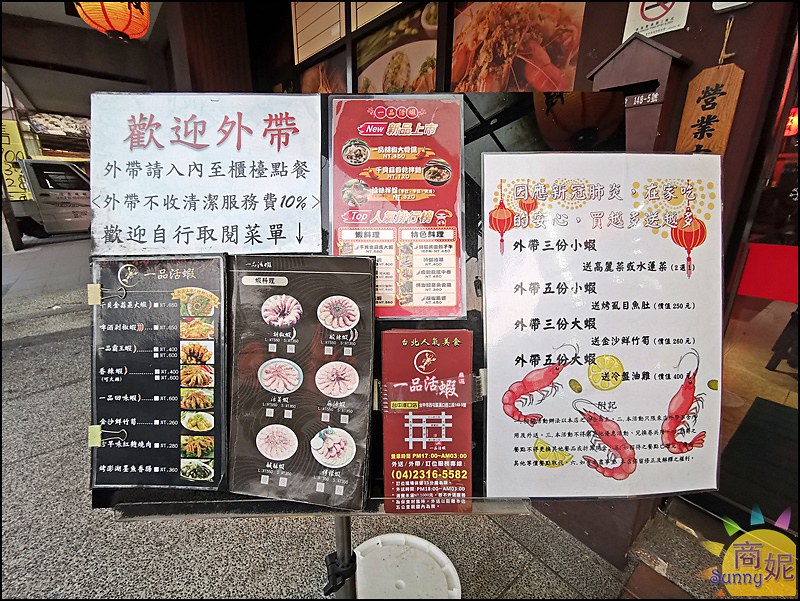This image captures a bustling outdoor food market area with an array of vivid details. The ground is paved with materials resembling gravel or granite. Several colorful posters and banners written in Chinese or Japanese are prominently displayed, showcasing a variety of food items, including red shrimp and assorted dumplings, with some having red or white backgrounds. In the upper part of the image, a yellow paper lantern is hanging to the left, adding a traditional touch to the scene. Visible through a window is a small white pickup truck, hinting that this area might be in an Asian country. The right bottom corner features a logo resembling a sun with multicolored rays and the word "Sunny" written in English, accompanied by Japanese text. Various structures and a concrete sidewalk complete the busy setting, highlighting it as a lively street food hub.